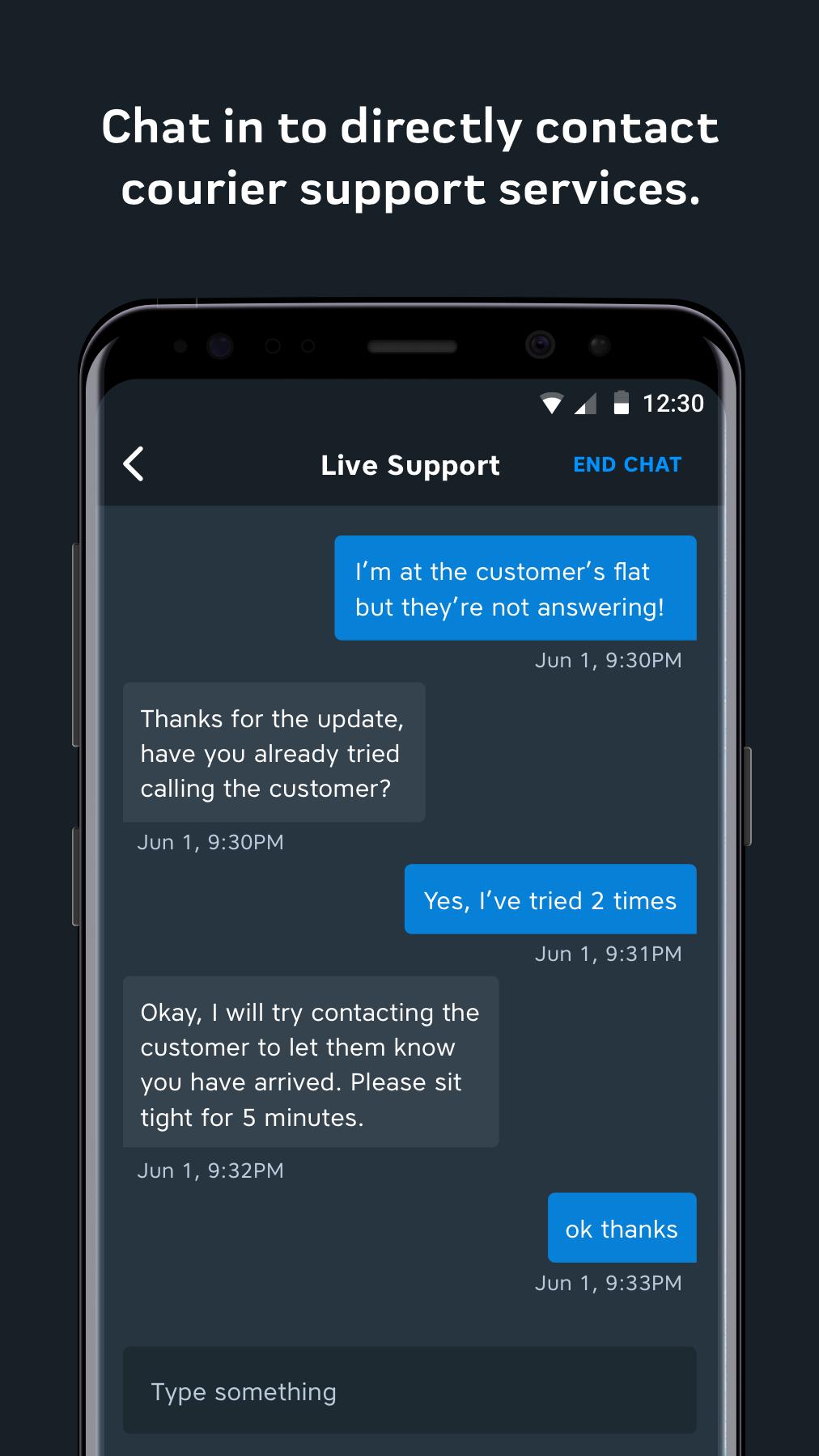The image displays a smartphone screen showcasing a web advertisement for a courier support service's live chat feature. The vertical, black screen prominently features bold white text at the top, stating "Chat in to directly contact courier support services." Below this heading, an image of a black smartphone is displayed to illustrate the service.

On the smartphone screen, the time shows 12:30, and the battery icon is at 50%. The top section of the phone screen features the text "Live Support" in white, with a bright blue "End Chat" option on the right-hand side.

The live chat exchange depicted on the phone is between a courier and a support representative. The courier's messages appear in a bright blue bubble with white text, while the support's responses are shown in white text on a black background. 

The conversation is as follows:
- At June 1st, 9:30 p.m., the courier sends a message: "I'm at the customer's flat but they're not answering."
- The support responds: "Thanks for the update. Have you already tried calling the customer?" also at June 1st, 9:30 p.m.
- The courier replies: "Yes I've tried two times."
- Support then answers: "Okay I will try contacting the customer to let them know you have arrived. Please sit tight for five minutes."
- The final message from the courier reads: "Okay thanks."

The exchange underscores the direct and immediate assistance available through the live support feature for couriers in the field.